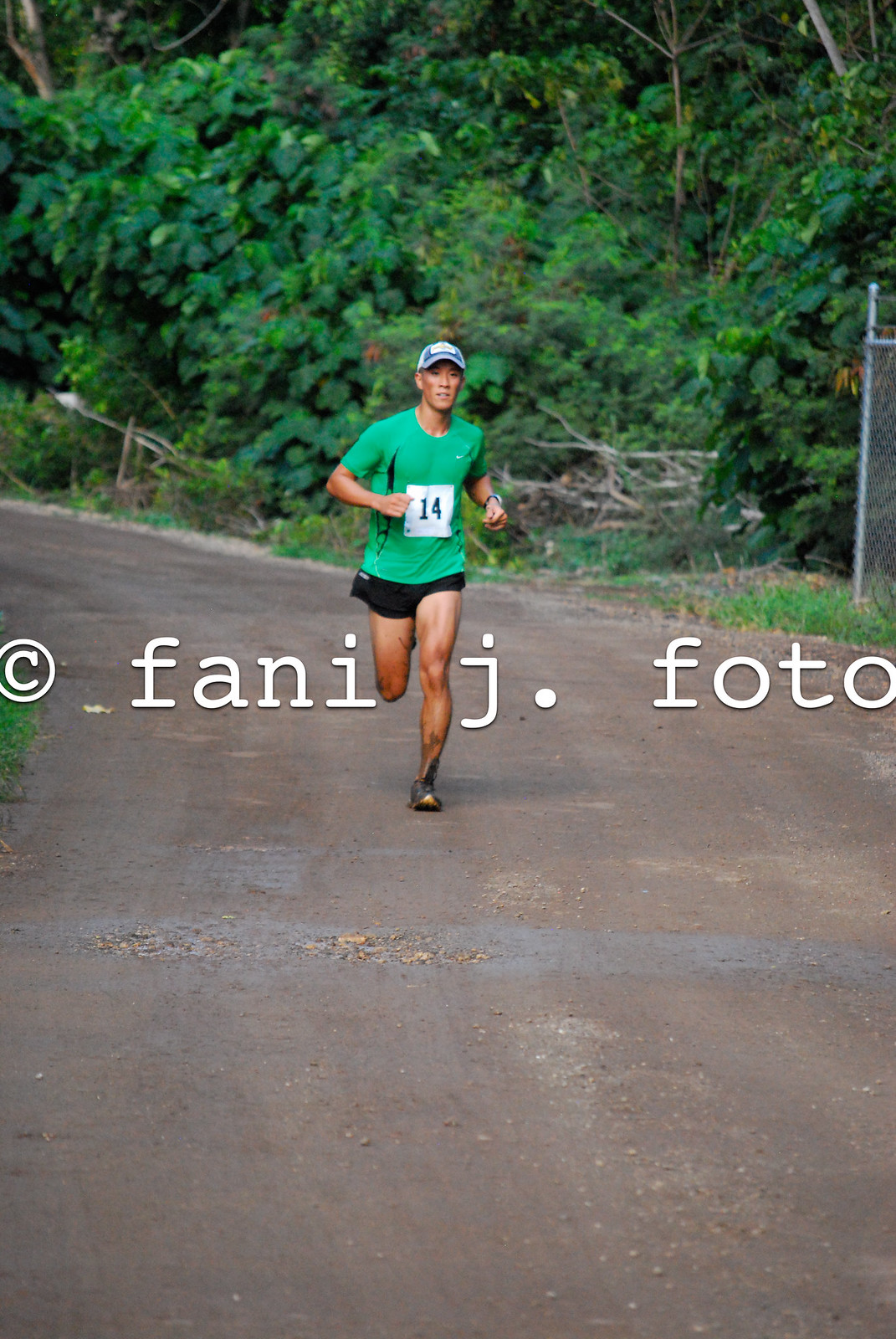The photograph captures an outdoor scene of a man running towards the viewer, likely participating in a race. He is clad in a green t-shirt with the race number "14" prominently displayed on a white square bib attached to his chest. He wears short black shorts and black sneakers with visible signs of wear. A dark blue baseball cap with a dark gray brim and a small white patch sits on his head. The man's skin tone is tan on exposed limbs and face, but appears paler on the upper legs. A fitness tracker or watch is visible on his wrist. The runner is navigating a slightly weathered gray pavement, which shows lighter and darker patches. The background reveals a lush, forested area with dense green foliage and intertwined branches, alongside a small visible portion of a gray chain-link fence to the right. The scene is bathed in daylight. A watermark text reading "© FANIJ.FOTO" is superimposed across the middle of the photo, partly obscured by the runner's legs.